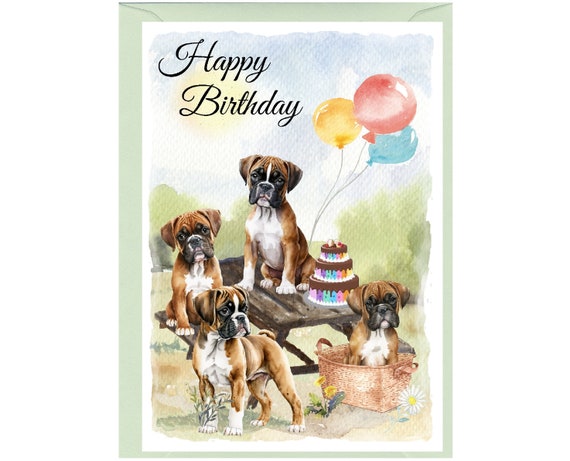This vertically aligned rectangular image depicts a charming birthday greeting card. The card rests atop a light greenish-gray envelope, slightly larger in size. Encapsulated by a white border, the card's watercolor illustration portrays a serene park scene with a pale yellow sun nestled in the upper left, surrounded by shades of blue sky. Sketched gray and white clouds gently float beside the sun. Centered in the scene is a dark brown wooden picnic table, adorned with a whimsical, multi-tiered cake decorated with brown trim. Four adorable puppies of boxer-like breed, characterized by their brown and white coats and black facial markings, animate the scene: one sits atop the table, another on the bench, a third within a wicker basket underneath, and the fourth stands nearby. Vibrant flowers emerge from the brown dirt and grass at the table's base, while colorful balloons—yellow, pink, red, and blue—float on three thin gray strings in the background. The upper left corner of the card showcases the phrase "Happy Birthday" elegantly scripted in black or dark brown cursive.